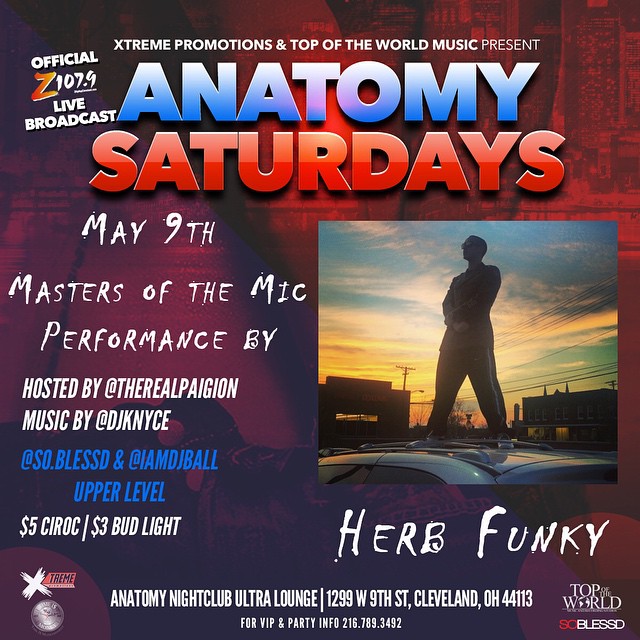This vibrant flyer, set against a dynamic background of dark red and purple, promotes an exciting event at the Anatomy Nightclub Ultra Lounge, located at 1299 West 9th Street, Cleveland, Ohio 44113. At the top, in striking white text, it announces, "Extreme Promotions and Top of the World Music present," followed by "Anatomy Saturdays" in large blue and red letters. The top left corner highlights an "Official Z107.9 Live Broadcast."

A central photograph captures a man standing on a silver car, dressed in a tracksuit and sunglasses, silhouetted against a vivid sunset with a blue sky and white clouds. The image enhances the edgy, nightlife vibe of the flyer.

The event, scheduled for May 9th, features a "Masters of the Mic" performance by Herb Funkey (H-E-R-B-F-U-N-K-E-Y). The proceedings are hosted by @TheRealPieGun, with music by @DJKNYCE, @so.blessed, and @IMDJBall. Attendees can enjoy $5 Ciroc and $3 Bud Light on the upper level.

The bottom of the flyer provides essential details for party-goers: "Anatomy Nightclub Ultra Lounge, 1299 West 9th Street, Cleveland, Ohio 44113. For VIP and party info, call 216-789-3492." Additionally, it promotes "Top of the World So Blessed" in varied text colors.